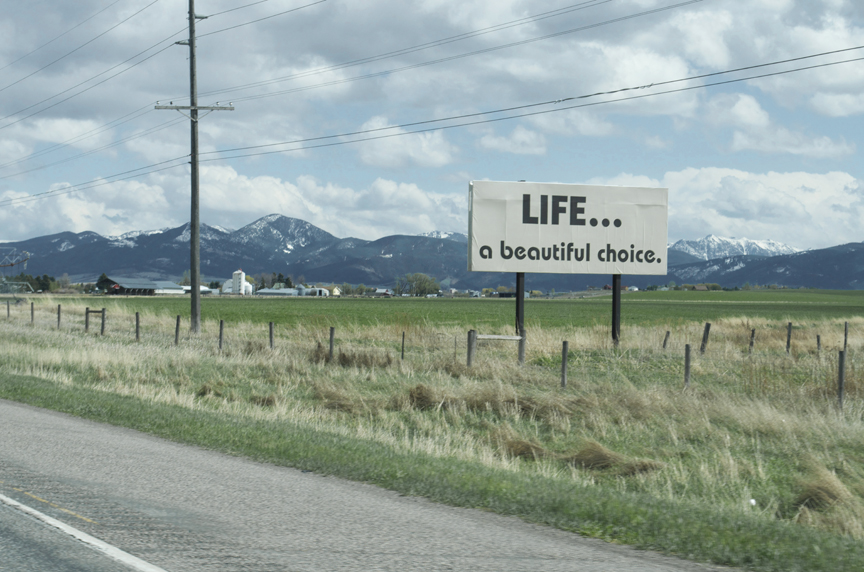An outdoor scene captures a tranquil suburban landscape. In the foreground, the edge of a road is visible, lined with a strip of grass that gently slopes into a field laden with hay. This field is enclosed by a simple wooden fence. Dominating the forefront is a white billboard on two sturdy wooden legs, bearing the phrase "Life... a beautiful choice" in bold black letters. In the mid-ground, a lone telephone pole stands calmly against the horizon. Farther back, several buildings, both white and dark, dot the landscape, signifying a small suburban area or a modest city. The background is framed by snow-capped trees under a vibrant blue sky, filled with a scattering of fluffy, white clouds.